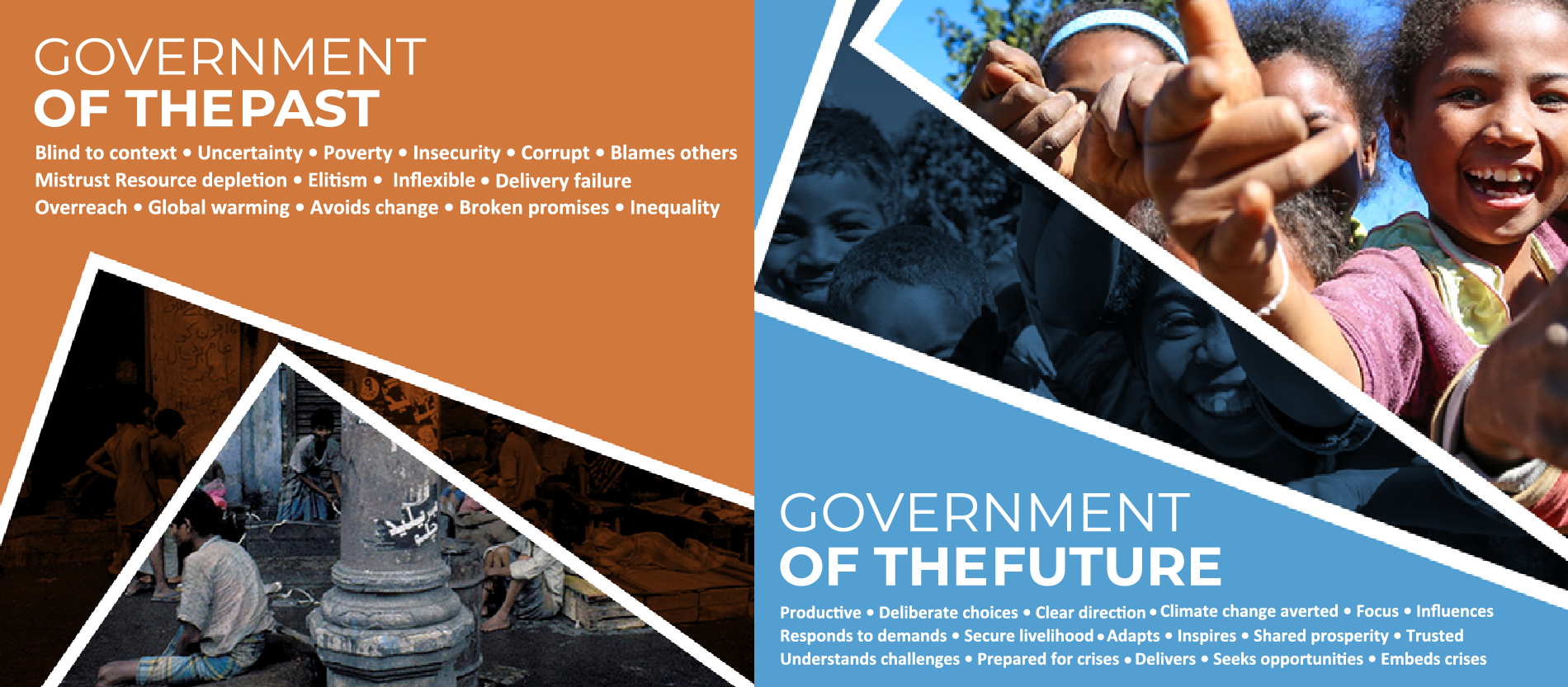The image appears to be a website or advertisement with a divided layout, presenting a stark contrast between two types of government. The left side of the image, marked by a brownish-orange background, is titled "Government of the Past" with a list of negative attributes in white text: Blind to Content, Uncertainty, Poverty, Insecurity, Corrupt, Blames Others, Mistrust, Resource Depletion, Elitism, Inflexible, Delivery Failure, Overreach, Global Warming, Avoids Change, Broken Promises, and Inequality. Below this text are bleak images of people sitting in dirt, columns, and impoverished areas. In contrast, the right side features a blue background titled "Government of the Future" with positive attributes like Productive, Deliberate Choices, Clear Direction, Climate Change Averted, Focus, Influences, Responds to Demands, Secure Livelihood, Adapts, Aspires, Shared Prosperity, Trusted, Understands Challenges, Prepared for Crisis, Delivers, Seeks Opportunities, and Embeds Crises. Above this text, a vibrant photo of happy, healthy children playing emphasizes a more hopeful outlook.